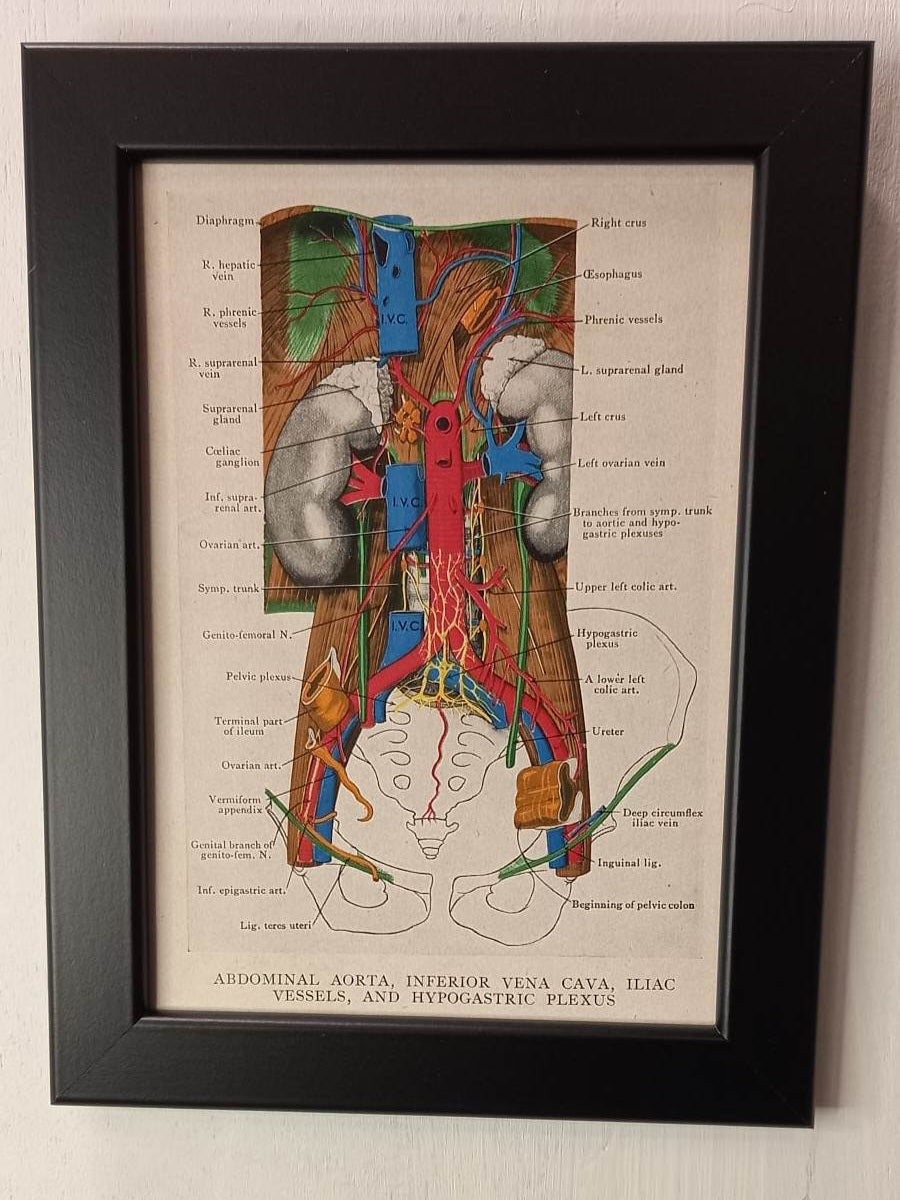This indoor photograph showcases a rectangular, dark brown or black wooden frame, affixed to a wall made of light brown or tan-colored wood paneling. Inside the approximately 5 to 6 inches high and 4 inches wide frame is a detailed anatomical diagram emphasizing the cardiovascular and abdominal systems, set against a light brown background. The diagram features a variety of human body parts rendered in multiple colors: the kidneys in grey, muscles in brown, arteries and veins prominently in red and blue respectively, and additional sections in various other hues. Accompanying the detailed illustration, all labeled parts and structures are identified with black text. Key anatomical parts included are the diaphragm, lungs, ovarian artery, and the hypogastric plexus, among others, outlined with lines extending to the respective labels. Notably, at the bottom of the diagram, written in capital letters, are "ABDOMINAL AORTA," "INFERIOR VENA CAVA," "ILLIAC VESSELS," and "HYPOGASTRIC PLEXUS," further emphasizing its focus on the human body's vascular and abdominal regions.